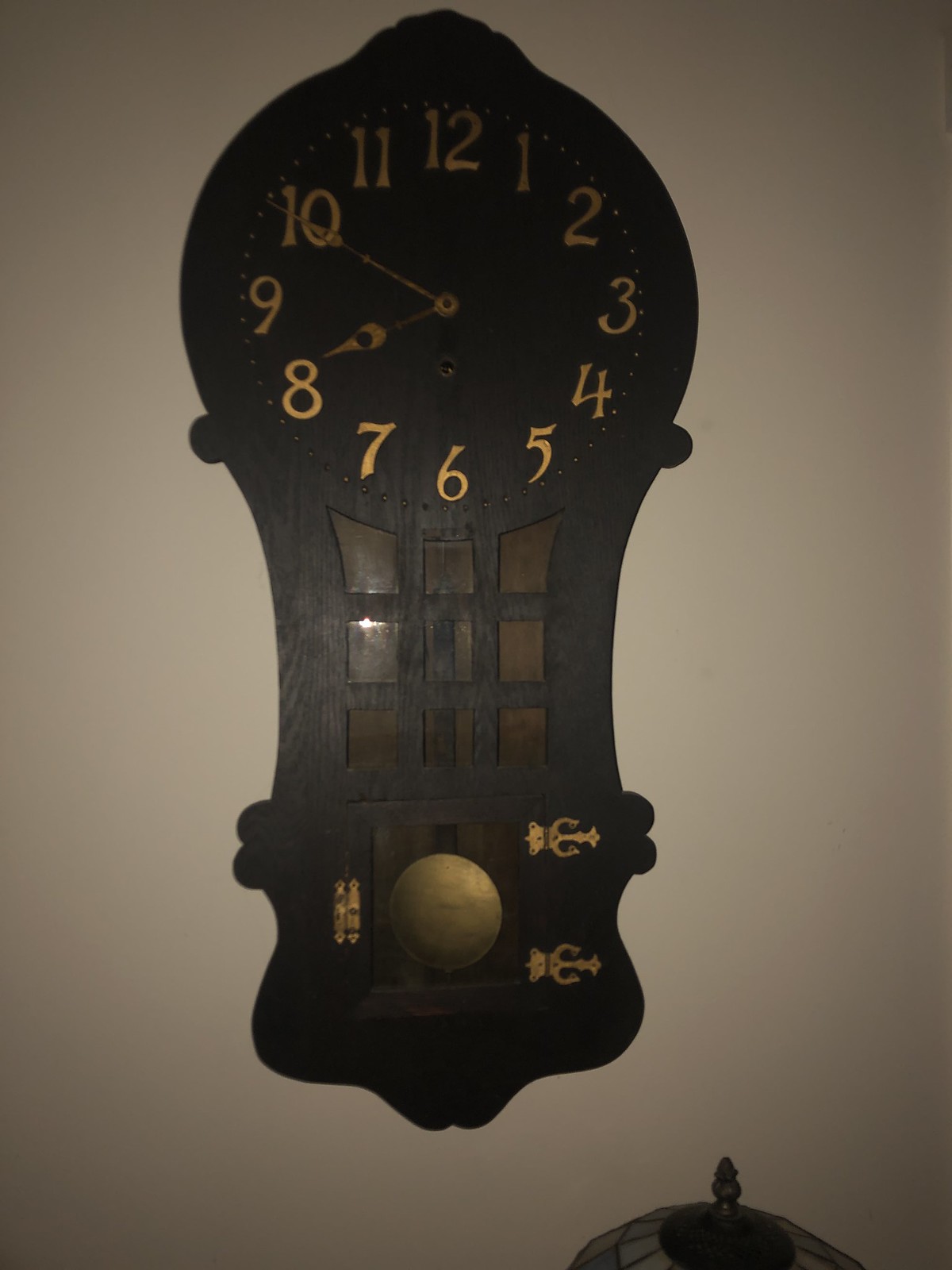The photo features a large, vintage wall clock made of dark wood, resembling a grandfather clock. It is mounted on a white wall. The clock face is circular with a slightly rounded top above the 12, creating a shape akin to a key. The numerals and delicate hands are golden, and they indicate that it is 10 minutes to 8 o'clock. Below the clock face, there are nine mini glass windows arranged vertically, revealing the internal mechanisms of the clock, including a prominent golden pendulum-like element. The lower part of the clock includes a small door with gold hinges. In the bottom right corner of the image, the tip of a vintage glass lamp with a stained glass lampshade is visible, and in the bottom left corner, a small portion of another lamp can be seen.